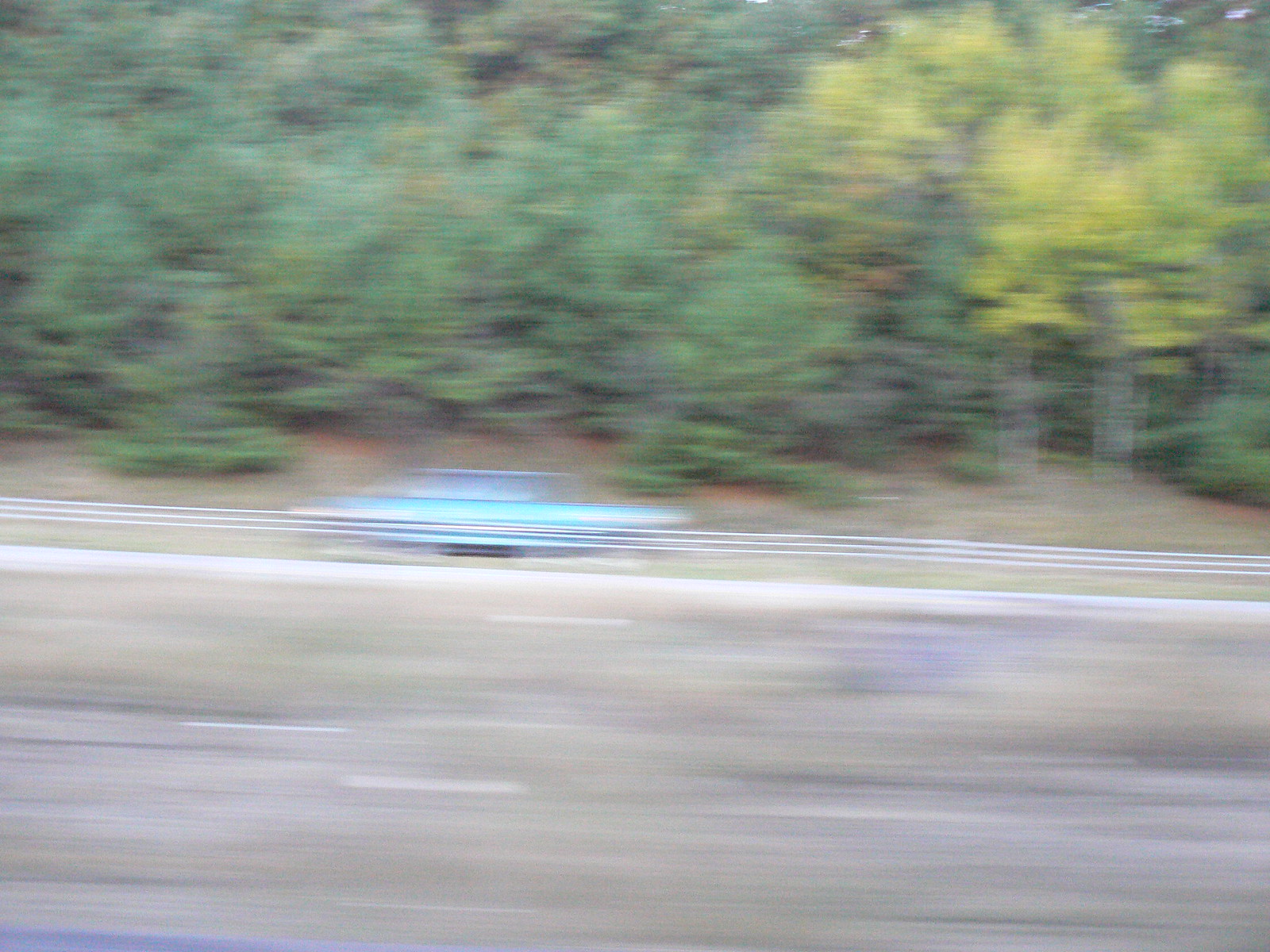This color photograph captures a very blurry image of a blue car traveling on a highway. The photograph appears to have been taken from a moving vehicle, resulting in the blurred effect. The highway runs diagonally across the page, slanting slightly. Positioned just left of center, the blue car appears to be an older model, heading up an incline on the right side of the road. To the right of the car, a tree line, featuring both dark green and light yellowish trees, sits atop a hill. A guardrail, likely acting as a divider between the two sides of the highway, cuts across the middle of the scene. The ground beneath the car has a sandy, light brown to off-white hue. The overall composition suggests a fast-paced, dynamic setting that rendered the image almost abstract due to the motion blur.